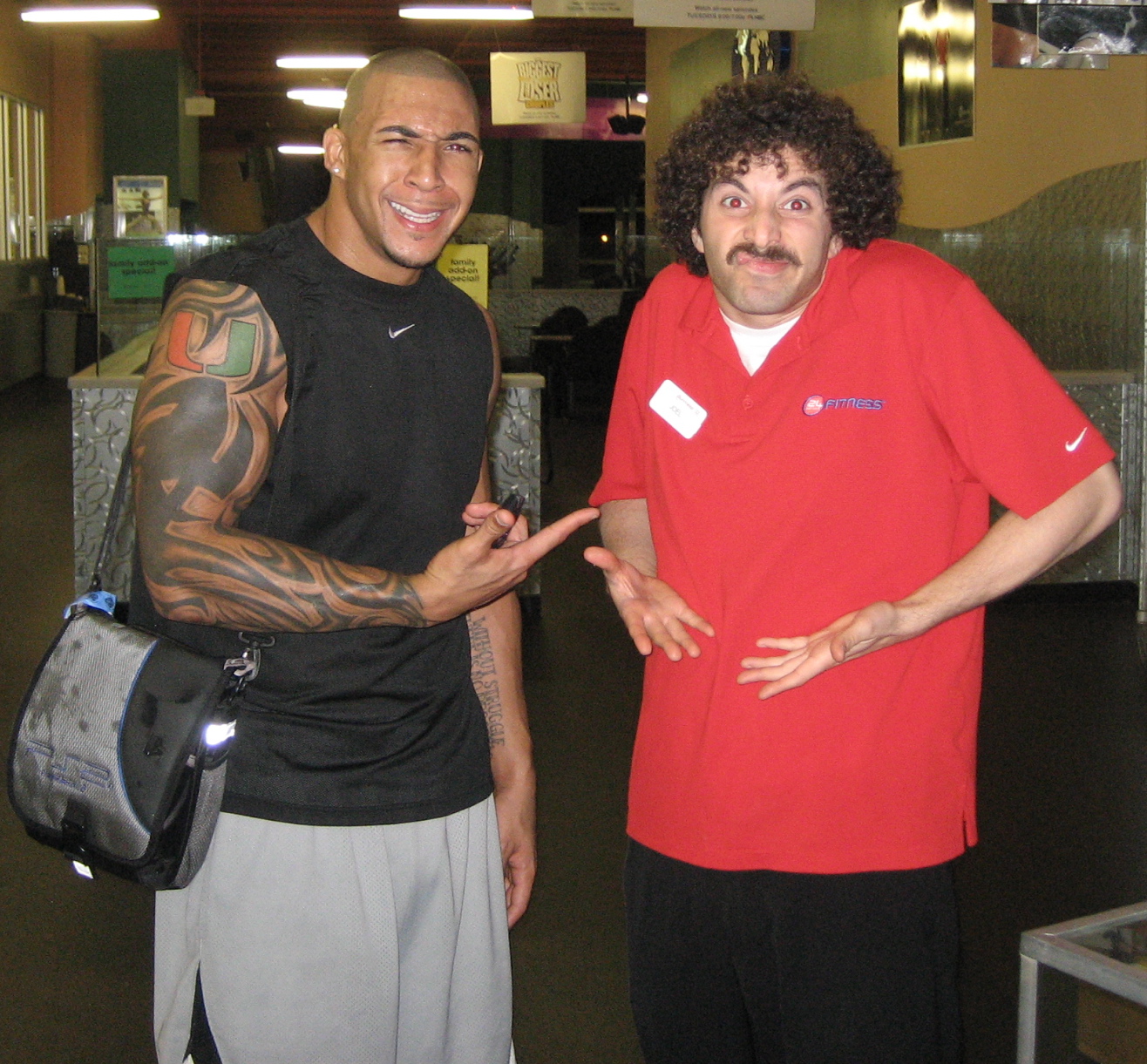In the photograph, two men stand side by side, each conveying distinct expressions. The man on the left is dressed in a black sleeveless t-shirt featuring a white Nike check mark near the neckline, paired with gray shorts that have a black stripe running down the sides. A black strap attached to a silver and black shoulder bag runs over his right shoulder, hanging down to the left. His appearance is further accentuated by tattoos visible on both arms, a closely shaved head, and dark eyebrows. He is mid-gesture, pointing towards the other man with his right arm bent at the elbow, his mouth partially open as if making a point, squinting slightly but with an amused expression.

The man on the right, shrugging with open palms and raised eyebrows, is dressed in black pants and a red polo shirt adorned with a white rectangular name tag on one side and a blue "24 Hour Fitness" logo on the other. The polo shirt, which also has the Nike logo on the arm, is worn over a white t-shirt with both buttons undone. He has very curly dark brown hair, a mustache, and an expression that suggests bewilderment as his shoulders are raised, giving the impression that he is asking a question or expressing confusion. His open hands add to this effect. The background features a mix of elements including a glass wall, counter space, and various objects, providing a subtle setting for the captured moment.